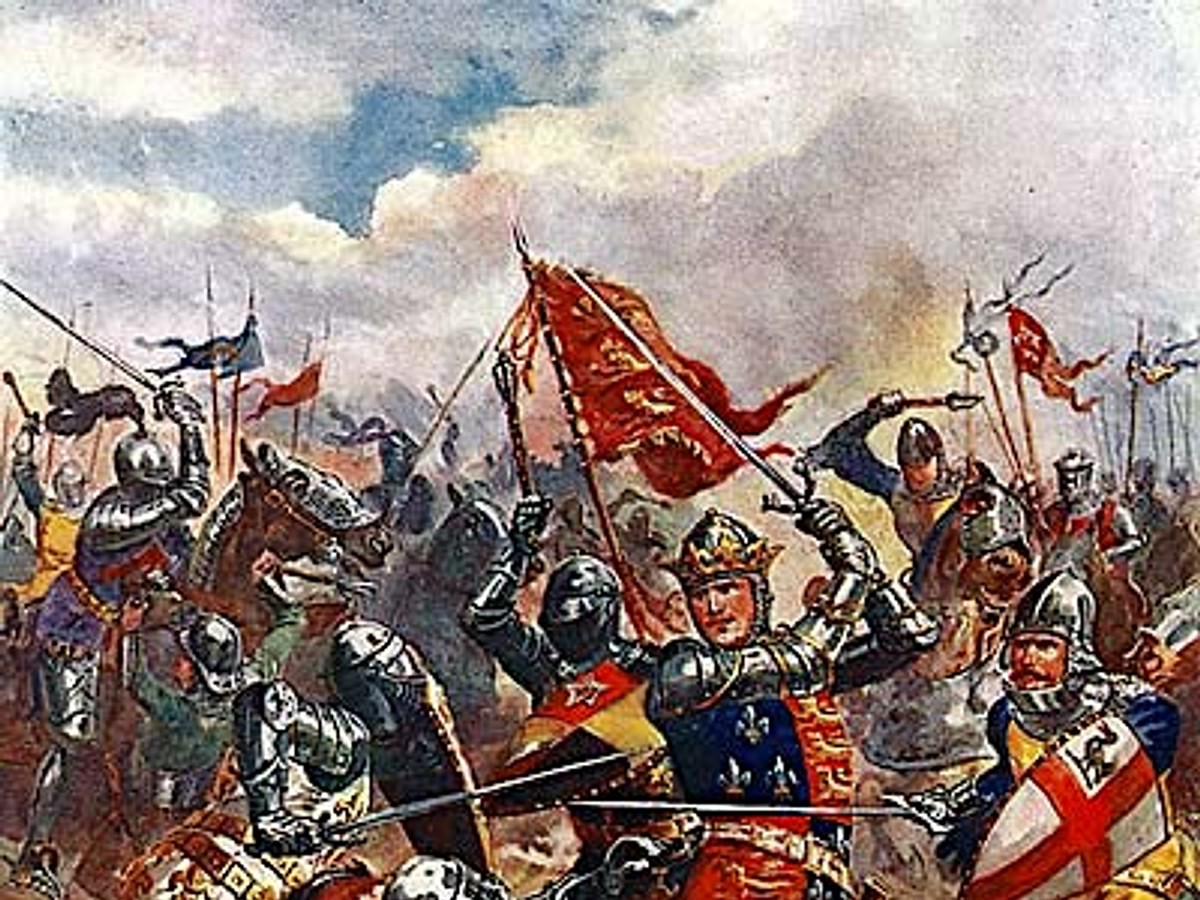This image is a vibrant, detailed painting capturing a chaotic medieval battle scene. The top half features a mostly cloud-covered blue sky, while the bottom half is filled with warriors in metal suits of armor. At the center of the composition stands a king, facing us directly, distinguishable by his gold crown and a long sword held aloft in both hands. His armor is adorned with a half-navy, half-red tunic featuring three fleur-de-lis. Around him, knights and soldiers, some on horseback and others on foot, engage in fierce combat. One noticeable detail includes a knight at the bottom with a white shield featuring a red cross. The chaotic scene is punctuated by bright, grainy watercolor tones of blue, red, white, and yellow, all outlined in black, with flags waving amidst the fray—particularly a tattered red flag with yellow or gold images, held high by a figure behind the king. The overall atmosphere is one of vivid and intense wartime struggle, set against the backdrop of a cloudy, gray sky.